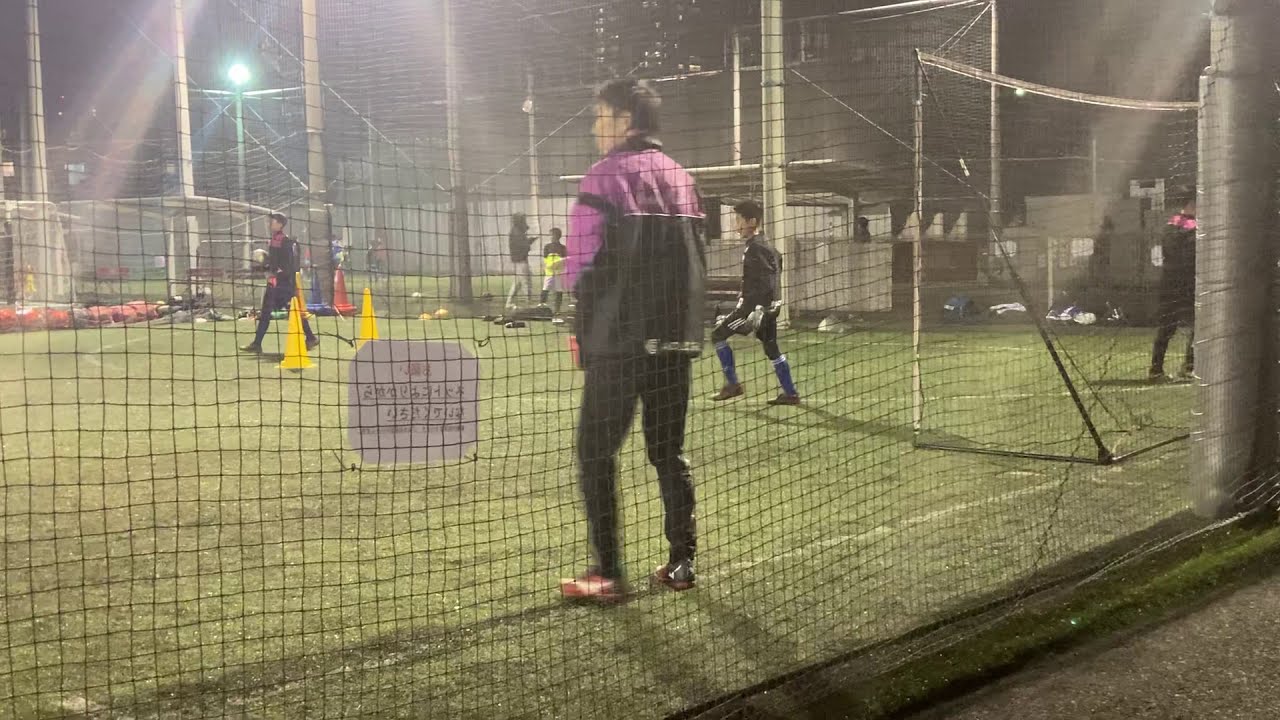This photographic image captures a nighttime soccer practice at an outdoor park. The scene is framed by soft, wavy plastic or fabric netting, placing the viewer just outside the practice area. Dominating the foreground is a man at the center wearing a purple and black jacket, black slacks, and distinct red sneakers. To his left, hanging on the mesh fence, is a sign adorned with Asian characters. In the mid-ground, a player dressed in a black jersey and pants holds a soccer ball as he moves leftward across the green field, accompanied by scattered yellow cones marking drills or boundaries. Further back, under the glare of brightly lit stadium-style lights, a few other players, including a visibly active goalie, engage in practice. The softly illuminated field contrasts with the darker silhouettes of single-story gray buildings and barely visible multi-story structures at the periphery. The entire scene imbues a sense of organized activity and cultural context within an East Asian setting.